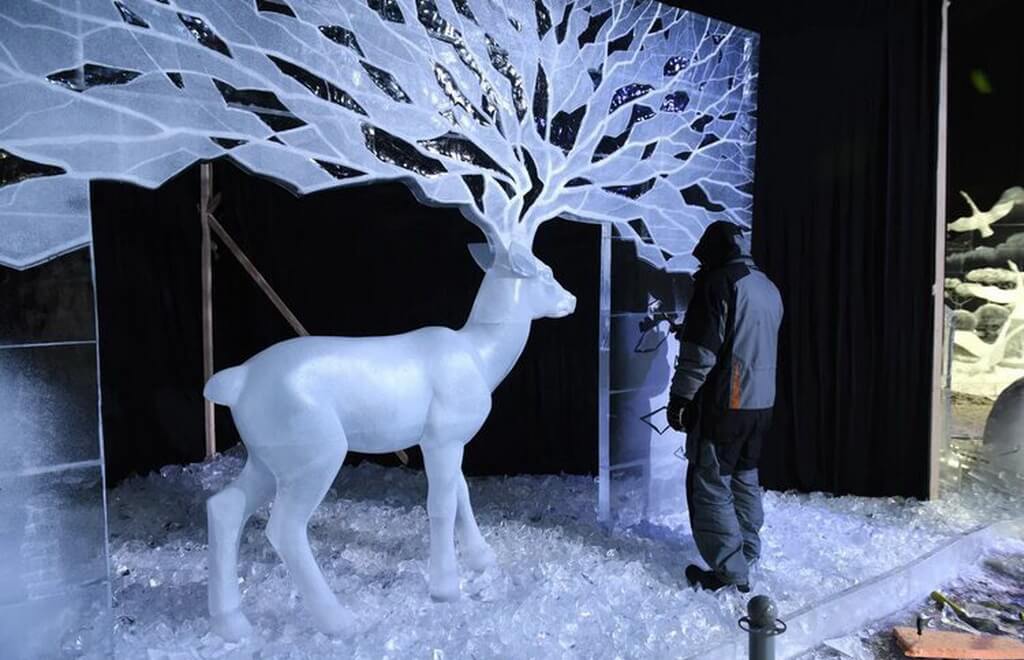The image captures an elaborate indoor scene resembling a museum exhibit with predominantly black walls. On the right side, there's a black barrier separating sections of the large room, partially enclosing a cream-colored mural depicting a bird flying with indistinct shapes below. A glass wall segment reveals a display of gray and brown rocks.

Dominating the scene, a striking ice-like sculpture of a deer with immense, intricate antlers extends towards the ceiling. The sculpture's design features an icy appearance interwoven with black accents. Emanating from the antlers are elaborate extensions resembling lightning bolts or branches with leaves, creating a dramatic visual effect.

The floor beneath the deer appears crystalline, mimicking the look of crushed ice or snow, enhancing the wintry ambiance. A man dressed in black and gray winter attire, with his hood up, stands near the sculpture, facing it. He holds what seem to be tools, possibly for carving, indicating he might be an artist or a technician attending to the exhibit. The photograph is a horizontal rectangle capturing this visually captivating tableau.